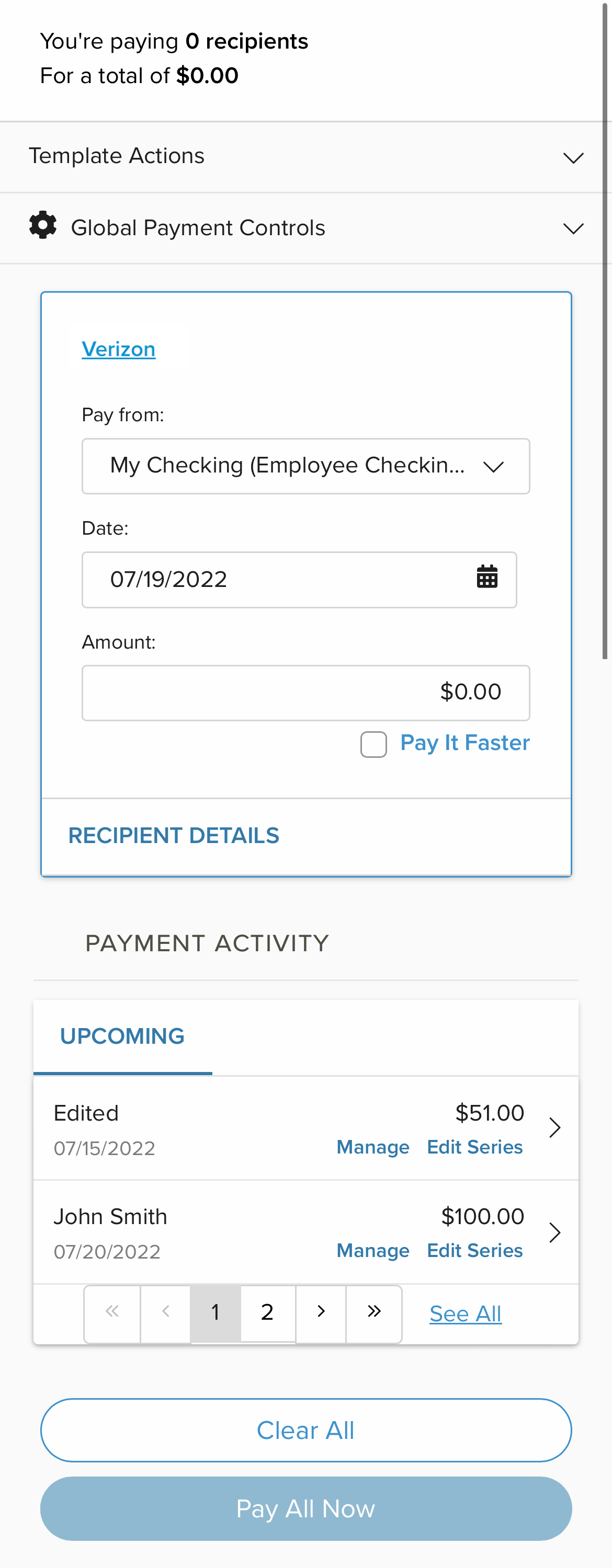Screenshot of a Payment Interface

---

The screenshot showcases a user-friendly payment interface dated July 19, 2022. The interface features various sections, including an option to pay from a checking account with designated fields for date and amount. 

Key Elements:

1. **Payment Input Section**:
   - **Date Field**: Allows users to select the payment date.
   - **Amount Field**: Currently shows an amount of $0.00.
   - **Recipient Details**: A button is available for inputting or viewing recipient details.

2. **Upcoming Payments**:
   - The list includes upcoming payments with relevant details:
     - **Edited Payment**: $51 scheduled for July 15, 2022.
     - **Payment to John Smith**: $100 scheduled for July 20, 2022.

3. **Options and Buttons**:
   - **Manage and Edit Series**: Provides options to manage and edit a series of payments.
   - **Clear or Pay All Now**: Buttons for clearing the current input or making all payments immediately.
   - **Past Payments and Activity**: Users can view all past payments and activities.

4. **Visual Cues**:
   - Sections such as "Upcoming Payments" and "Manage and Edit Series" are highlighted in blue, indicating they are clickable for further actions.

5. **Additional Details**:
   - There's a dropdown menu labeled "Pay from my checking, employee checking account," allowing users to select the desired account for payment.

The layout is straightforward, facilitating ease of use for payment planning. It hints at the user's potential effort to add Verizon to their payment list, although this is not certain.

The interface’s clear design aids in efficiently managing and scheduling payments.